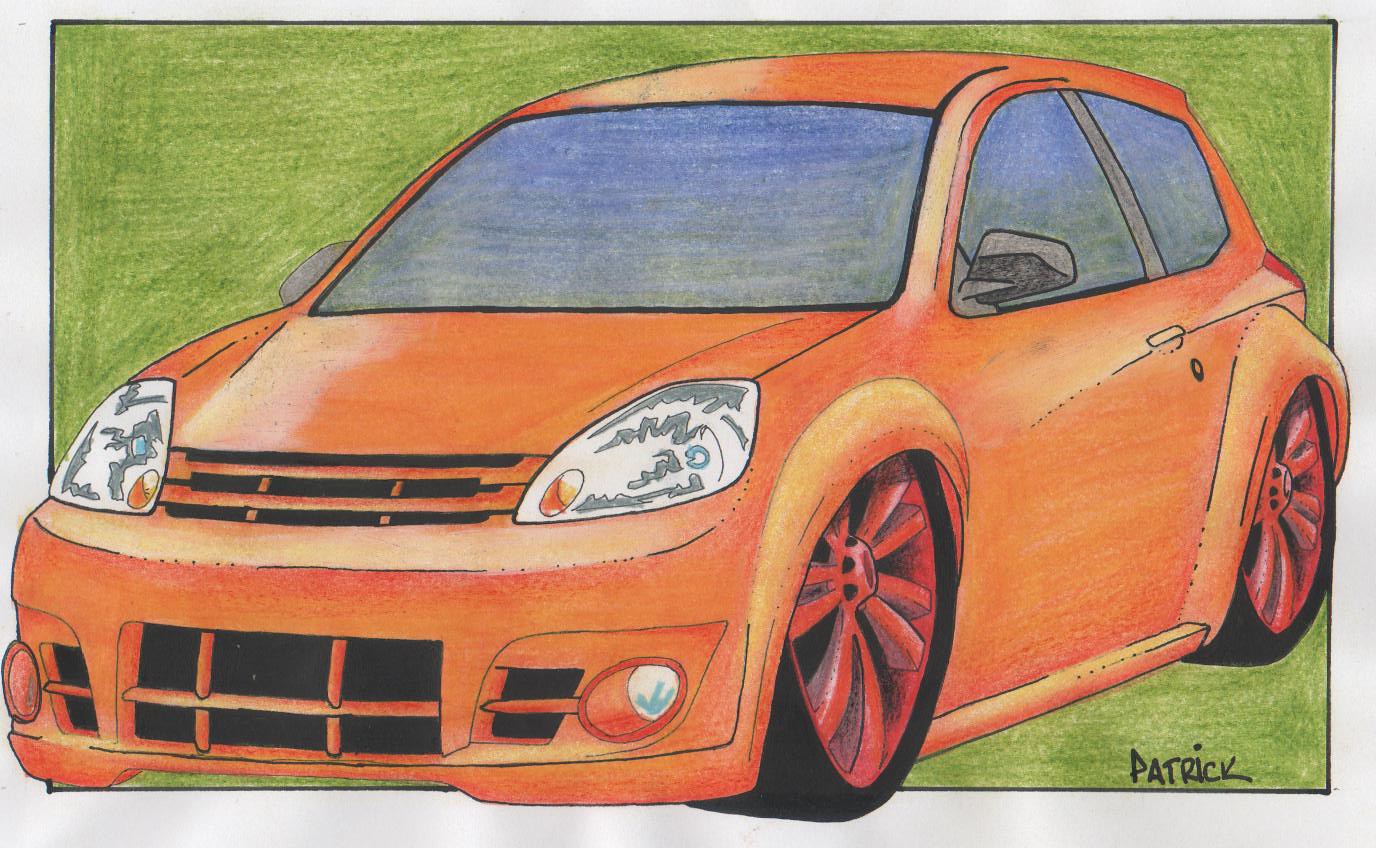The image depicts a detailed drawing of an orange hatchback-style sedan. The artwork is framed within a dual border: an inner black rectangle and an outer white margin. The scene's background is filled with a light green shading, creating a contrast with the vibrant car. In the bottom right-hand corner, the name "Patrick" is written in black letters. The front of the car extends beyond the black border, encroaching into the white outer margin, giving a sense of movement and dynamism. The car's headlights are highlighted with a silver hue, while its single door and sleek design are prominently featured. The rims are painted red, complementing the black tires. The windshield and windows display a bluish tint, adding a touch of realism to the illustration.